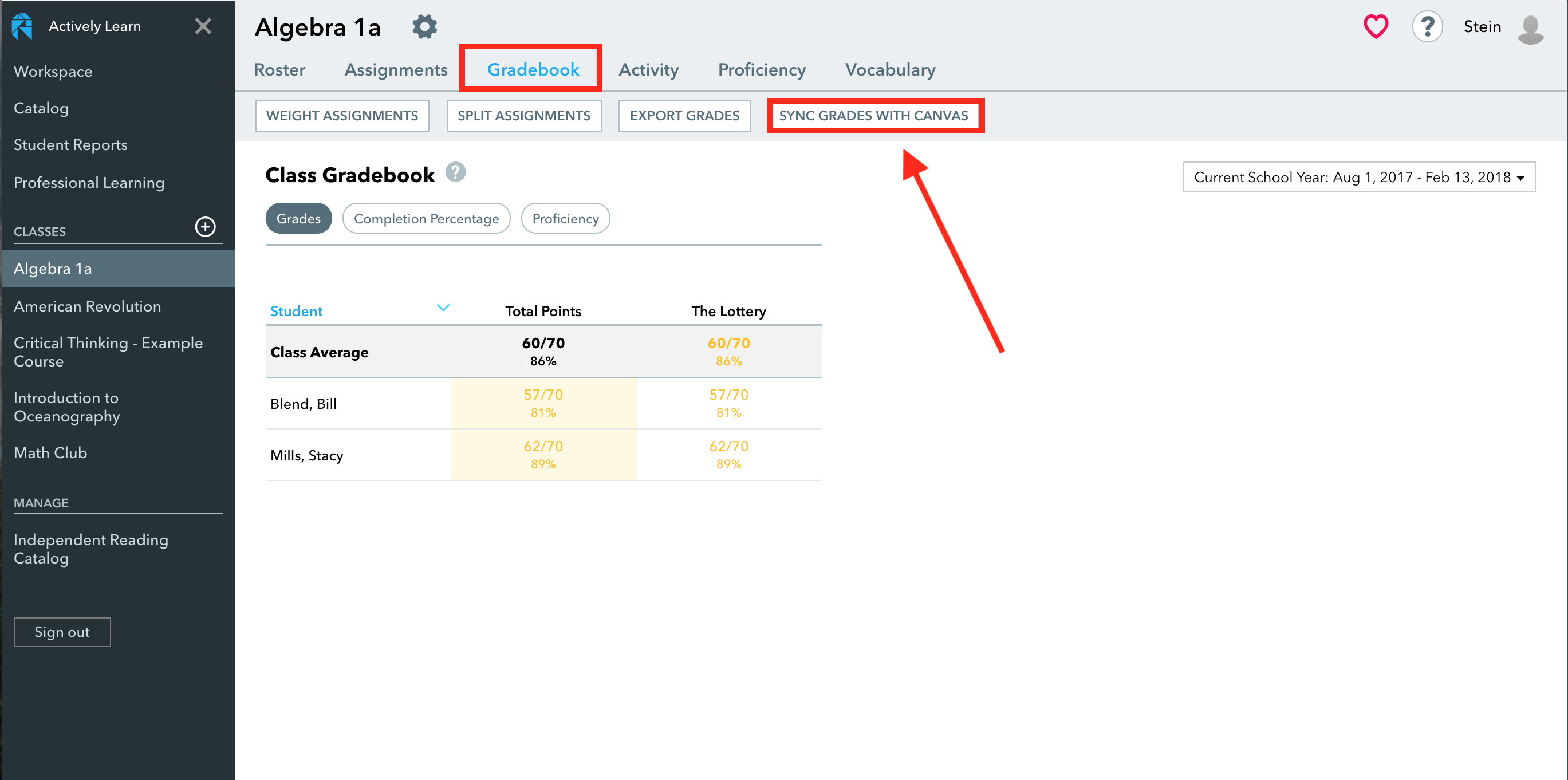The screen captures a detailed interface of the "Actively Learn" educational platform with a focus on the Algebra 1A course. At the top, the site header reads "Actively Learn" with a close button (X) next to it. 

A black navigation bar runs vertically down the left side of the interface, featuring several white-labeled tabs: Workplace, Catalog, Student Reports, Professional Learning, Classes, Algebra 1A, American Revolution, Critical Thinking, Example Course, Introduction to Oceanography, Math Club, Manage, Independent Reading, Catalog, and Sign Out. The "Algebra 1A" tab is highlighted, reflecting the currently active course.

At the top of the main content area, there are several gray tabs: Roster, Assignments, Gradebook, Activities, Proficiency, and Vocabulary. The "Gradebook" tab is selected, indicated by its blue color and a red box around it.

Below the main tab row, a secondary group of buttons includes options for Weight Assignments, Split Assignments, Export Grades, and Sync Grades with Canvas. These buttons are also highlighted with a red box and a red arrow pointing towards them, likely as part of a tutorial.

The main content area under these controls displays a section labeled "Class Gradebook," featuring columns for Grades, Completion Percentage, and Proficiency. Additionally, it lists students’ names, total points, and details. The class average is prominently shown below this table, stating a score of 60 out of 70, equating to 86%.

This comprehensive capture serves as a visual guide for users to navigate and utilize the grading features within the "Actively Learn" platform for the Algebra 1A course.